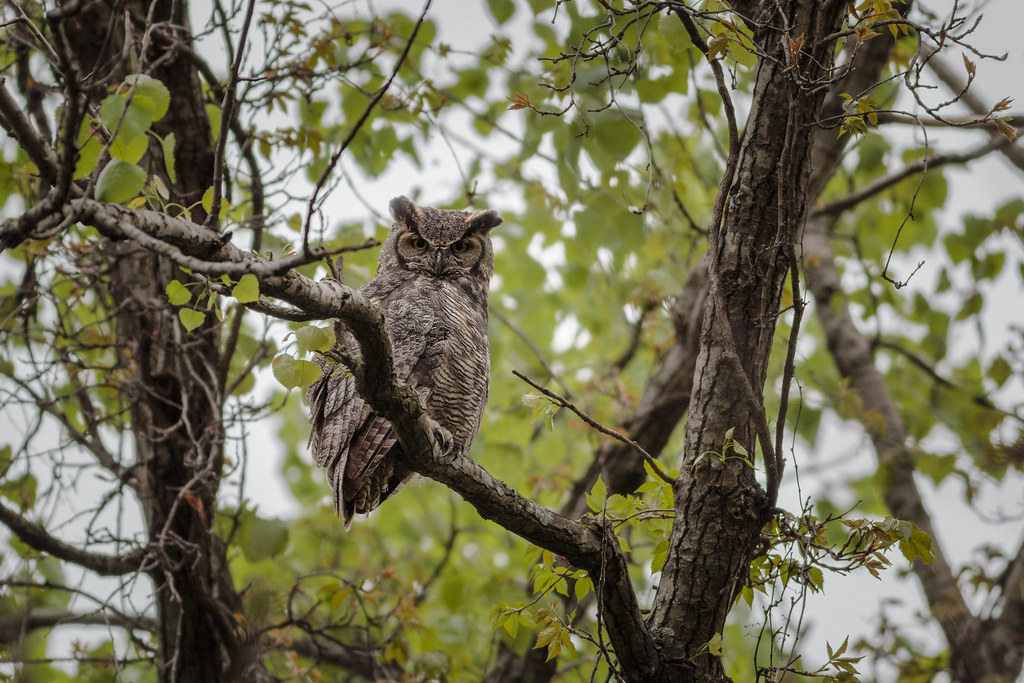This photograph captures a serene outdoor scene beneath a solid gray sky, offering a striking contrast to the lush greenery. Dominating the foreground is an intricate network of brown tree branches, their rough bark adorned with cracks and ridges that add texture to the image. Sprouting from these larger limbs are smaller branches, all adorned with a profusion of vibrant green leaves, creating a verdant canopy.

Nestled on one prominent branch in the foreground, an owl, with its brown feathers blending seamlessly with the tree, gazes directly at the camera. Its piercing eyes and determined expression give the impression that it stands vigil over its arboreal domain. In the background, another tree adds depth to the scene, its main branch jutting out at a crooked angle, breaking the symmetry and adding a layer of complexity to the composition. Together, these elements form a compelling tableau of nature's quiet strength and beauty.